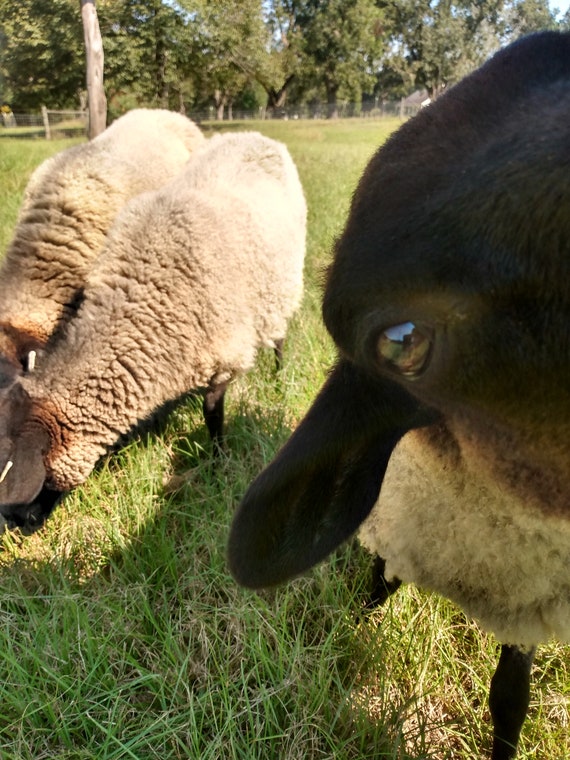In a sunlit afternoon scene, this photograph captures a trio of sheep amidst a picturesque pasture. The sky is a brilliant blue, and in the background, a line of trees stretches across the horizon with a glimpse of a low fence visible. The grass, lush and tall, measures about six to eight inches in height. Two of the sheep, with dark legs and tan wool, are engrossed in grazing on the left side of the frame. Meanwhile, the third sheep is positioned extremely close to the camera on the right, offering an intimate view of its eye and ear, which, at first glance, might be mistaken for a different animal's bill. This up-close sheep playfully gazes into the lens, contrasting with its oblivious companions. The sun illuminates the scene from behind, casting shadows in the foreground and enhancing the pastoral tranquility of the setting.